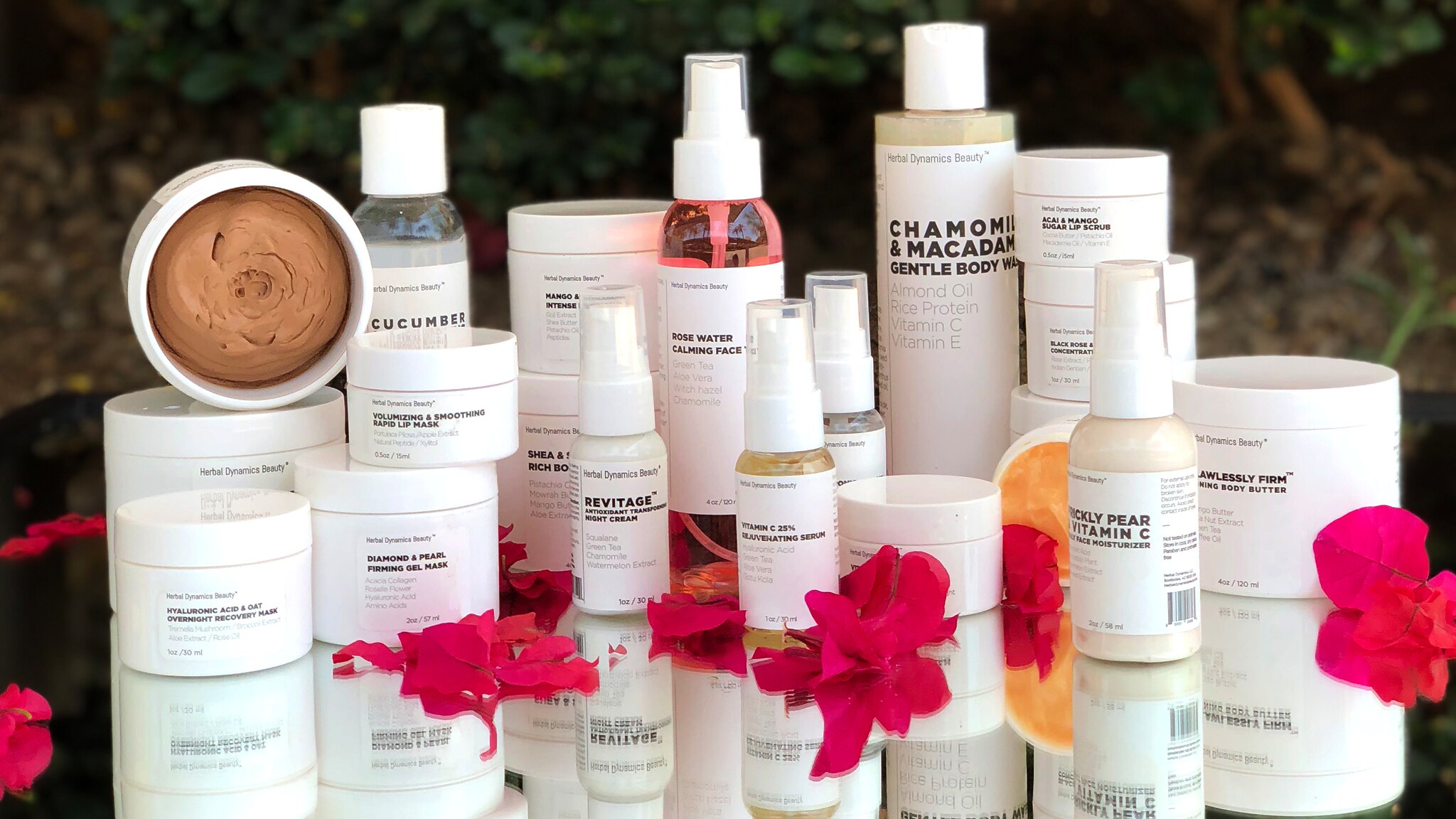A collection of cosmetic products from Herbal Dynamics Beauty is elegantly displayed on a mirrored tabletop. The assortment includes predominantly white jars with screw lids, complemented by a few tall, clear spray bottles. Each product features a minimalist design with stark, all-white labels and small, sans-serif font that is somewhat difficult to read. Despite this, several product names are discernible: a clear bottle labeled with "cucumber," a jar for "Volumizing and Smoothing Lip Mask," "Diamond and Pearl Firming Gel Mask," "Prickly Pear Vitamin C Moisturizer," "Flawlessly Firm Body Butter," and "Chamomile and Macadamia Gentle Body Wash."

The scene is enhanced by the scattering of pinkish-red flower petals across the mirrored surface and around the bottles and jars, adding a touch of color and elegance to the display. The background is subtly blurred, showcasing green foliage that brings a natural, serene contrast to the otherwise stark and minimalist aesthetic of the products.